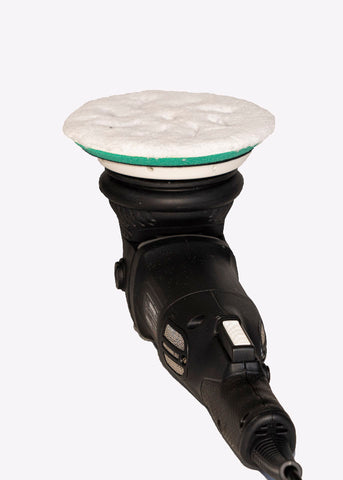The image vividly captures an electric buffer or waxer, positioned centrally against a stark white background. The tool, predominantly black, is turned handle-up, showcasing its underside. Attached to the bottom is a circular white pad with a green stripe, indicating its likely use as a buffing or waxing surface rather than traditional sandpaper. The soft appearance of the pad suggests it's designed for polishing surfaces, such as car bodies or furniture. A white switch can be seen on the tool, and the cord, barely visible, extends from the lower right side. The image is clear and well-lit, emphasizing the details and texture of the buffer. No additional objects, text, or labels are present to distract from the main subject.